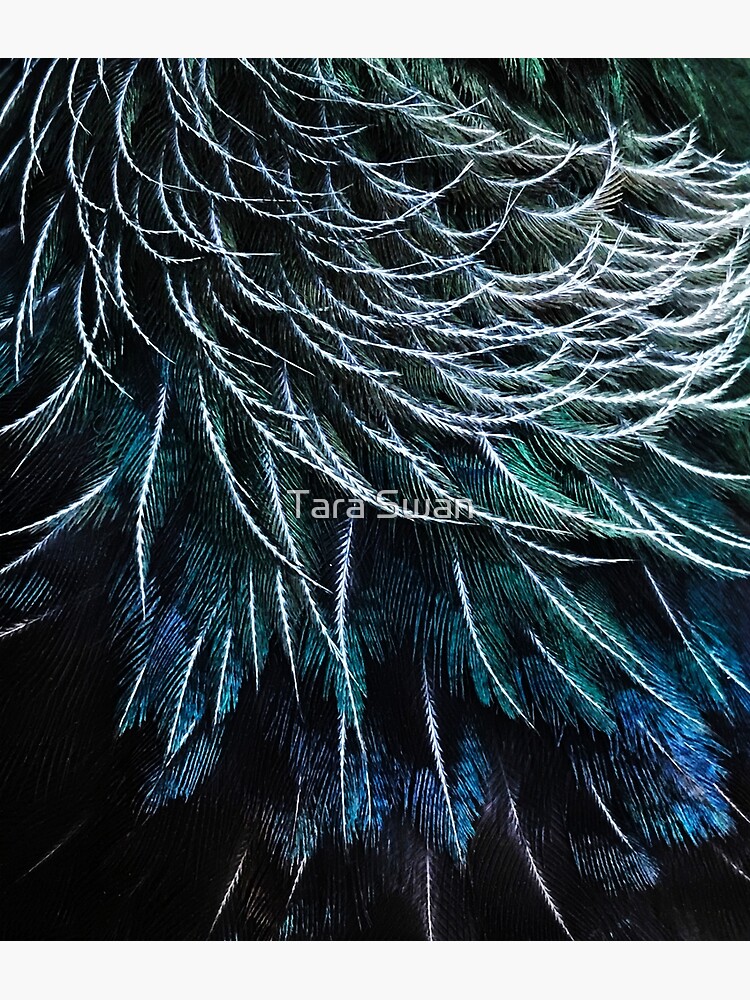The image is a detailed illustration of a spruce tree, focusing closely on its long, flowy needles. The branches, adorned with these needles, transition in color from green at the top to blue and then purple towards the bottom, with the edges at the very bottom shading into black. Amongst the branches, thinner white strands, resembling delicate stems, blow gracefully in the wind, giving an ethereal feel to the scene. The overall effect is realistic, despite the depiction being a drawing rather than a photograph. In the center of the illustration, the name "Tara Swan" stands out in semi-transparent white text, likely indicating the artist's signature.